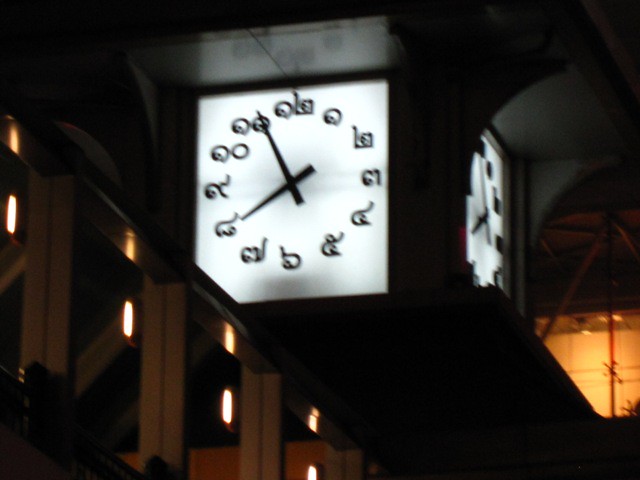A captivating nighttime photograph showcases an intriguing cube-shaped clock. Each side of the cube, excluding the top and bottom, is adorned with a clock face. The focal point of the image is the clock face on the front, which stands out with its white background and black hands. Instead of traditional numbers, the clock features unique black characters that suggest a different language. To the right, another clock face is partially visible but slightly blurred and out of focus, appearing to share the same design as the main one.

The photograph captures the ambiance of the night with multiple windows visible in both the foreground and background. These windows reflect an array of bright, orange-hued lights, adding a warm glow to the scene. The primary color palette of the image consists of stark contrasts between black and white, complemented by the varied yellow and tan tones emanating from the lights. This interplay of light and shadow brings a sense of depth and intrigue to the composition.